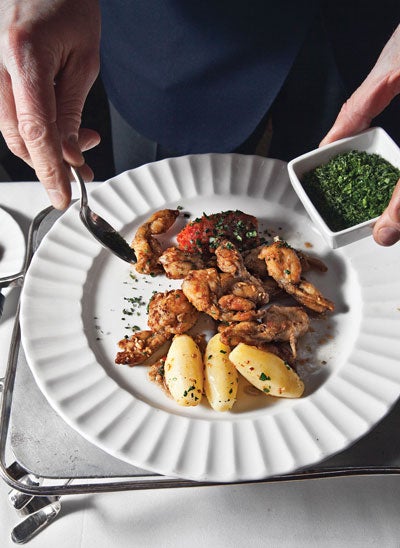An overhead photo captures a chef finishing a dish on a circular white plate with a ridged, thick rim. The center of the plate features three thin, skinned fingerling potatoes arranged at the bottom, accompanied by oblong pieces of what appears to be either chicken or peeled garlic, possibly mistaken for shrimp or scallops due to their unusual shape and brownish color. These pieces are garnished with finely chopped green herbs, likely cilantro. The plate, resting on a silver tray with feet, sits atop a white table. The top portion of the image reveals the chef, dressed in a blue shirt. Both hands are visible: the left hand holds a small, square dish containing the green herbs, while the right hand hovers a spoon above the plate, sprinkling the herbs over the dish.